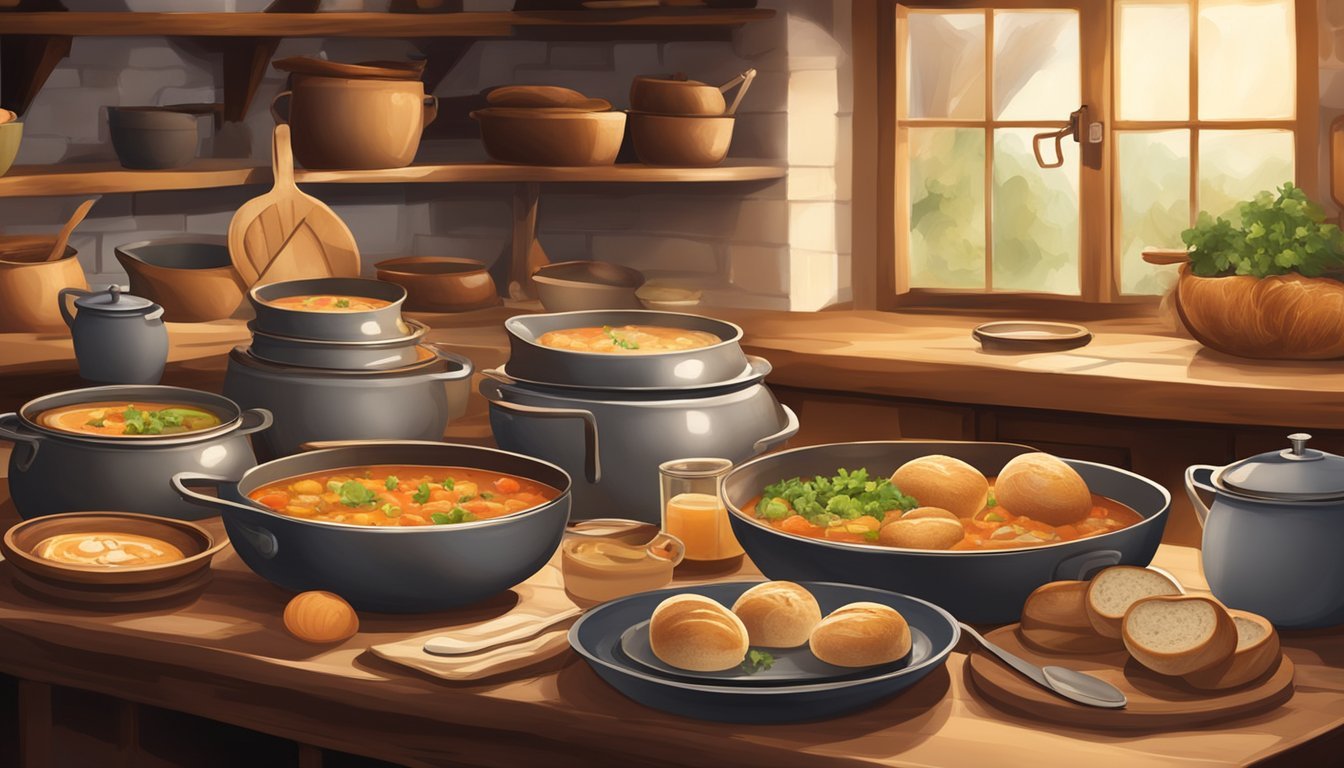The AI-generated image portrays a rustic, country-style kitchen, digitally rendered with notable imperfections and artifacting. At the forefront, a beautifully sanded, wooden table occupies the bottom of the image, laden with various kitchenware and food items. Dominating the scene are multiple gray metal pots filled with a striking orange liquid, possibly a stew or broth, garnished with green leaves on the surface. Among these pots, some overlap awkwardly due to the artifacting, creating the appearance of pots inside pots. Scattered around the table are wooden and metal vessels, alongside beautifully puffy rolls of bread, some of which rest on a cutting board to the right, while others float in the stew. A gray jug sits prominently on the right, adjacent to a wooden plate also holding bread. The backdrop features a gray brick-patterned wall, a defining characteristic of the earthy ambiance.

To the right, there's a double glass window with brown frames, casting light on the scene, while below it, a wooden countertop extends along the wall. The left side of the image showcases curved walls adorned with wooden shelves, holding a collection of mostly brown vessels. Near these shelves, a brown pot with lush green leaves adds a touch of natural beauty. Overall, it’s a detailed and inviting depiction of a cozy and culinary-rich rustic kitchen, despite the noticeable digital anomalies.